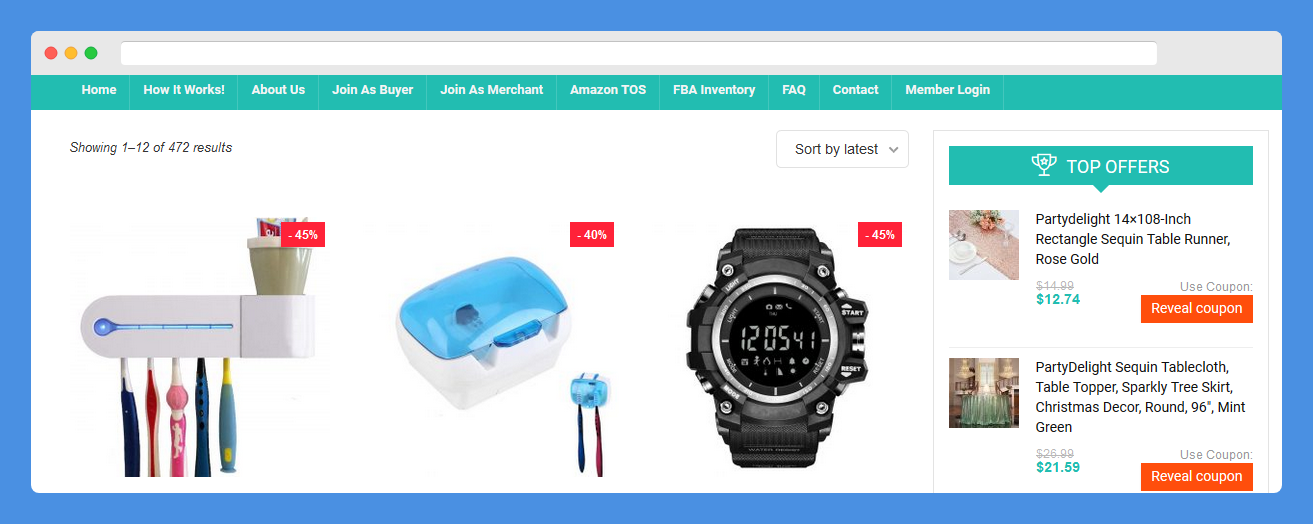The image shows a website page with a distinctive layout featuring three colored dots—red, gold, and green, positioned in the top left corner. This indicates where you typically close, minimize, or maximize the window. 

At the top, there is a search bar without any visible search key or button. Below this, several images of various discounted items are displayed. Notably, there are toothpaste brushes hanging, prominently marked with a banner stating they are 45% off. Adjacent to these hangs a white box with a clear blue lid, likely containing more toothbrushes, which are shown as 40% off.

A grey digital watch, reminiscent of a diver's watch with visible seconds, also appears in the lineup, prominently advertised as being 45% off.

Additionally, the website highlights its top offers, including a "Party Delight 14 by 108 inch rectangle sequin table runner" in rose gold. Another featured item is a "Party Light sequin table topper sparkly tree skirt Christmas decor," described as round with a 96-inch diameter in mint green. Both of these items have an option to "reveal coupon" through an orange clickable button for potential discounts.